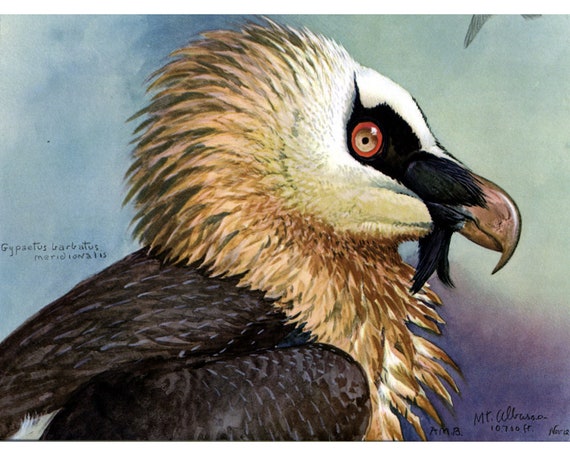This detailed painting or illustration prominently features a hawk, referred to as Gypsitus carcharatus meridius, presented in a side profile with much of its body and part of its wing visible. The hawk has striking plumage: its body feathers are a deep brown or almost black hue, while the feathers from the back of its head, around its neck, and down its chest are a distinctive gold or tan color. Its face is primarily white, accentuated by a bold black streak extending from its eye down to its large, sharp, brown beak, which has a pronounced hook at the tip. The bird's eye is brown, encircled by a vivid red ring, and two black feathers hang from the corners of its mouth, resembling a mustache. The background mixes gentle shades of blue and purple, adding depth to the composition. To the left of the bird is a script, possibly indicating the species name, and a signature at the bottom reads Mr. Williams.